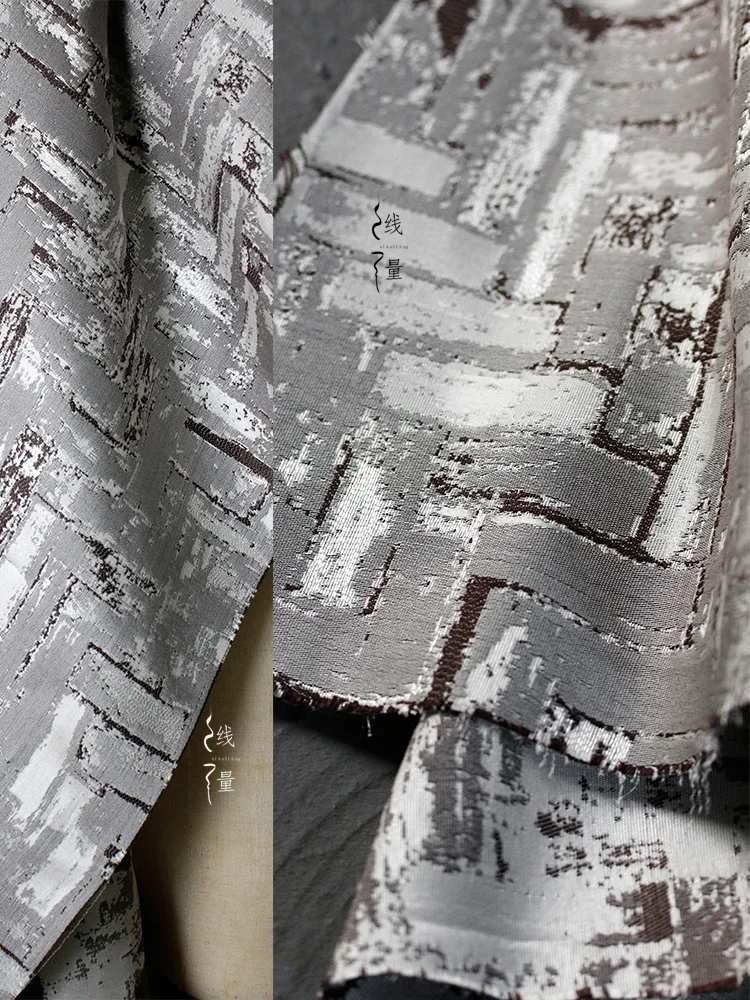The photograph is a close-up color image showcasing a piece of fabric with a herringbone pattern. The fabric alternates between tones of gray and white, with some dark brown spots that add a touch of variegation. It appears textured, almost as though the lines and bars were painted with a rough brushstroke, accentuating the weaved, rugged appearance. The fabric is divided into two sections, with the left section being narrower than the right. There are frayed threads hanging down at the bottom, suggesting that the fabric has been torn or worn over time. Situated on the left side of the image, there are small Chinese characters in white, which appear to function as a stamp or symbol, although they are not very prominent. The background is absent, ensuring that full emphasis remains on the detailed texture and intricate pattern of the fabric.